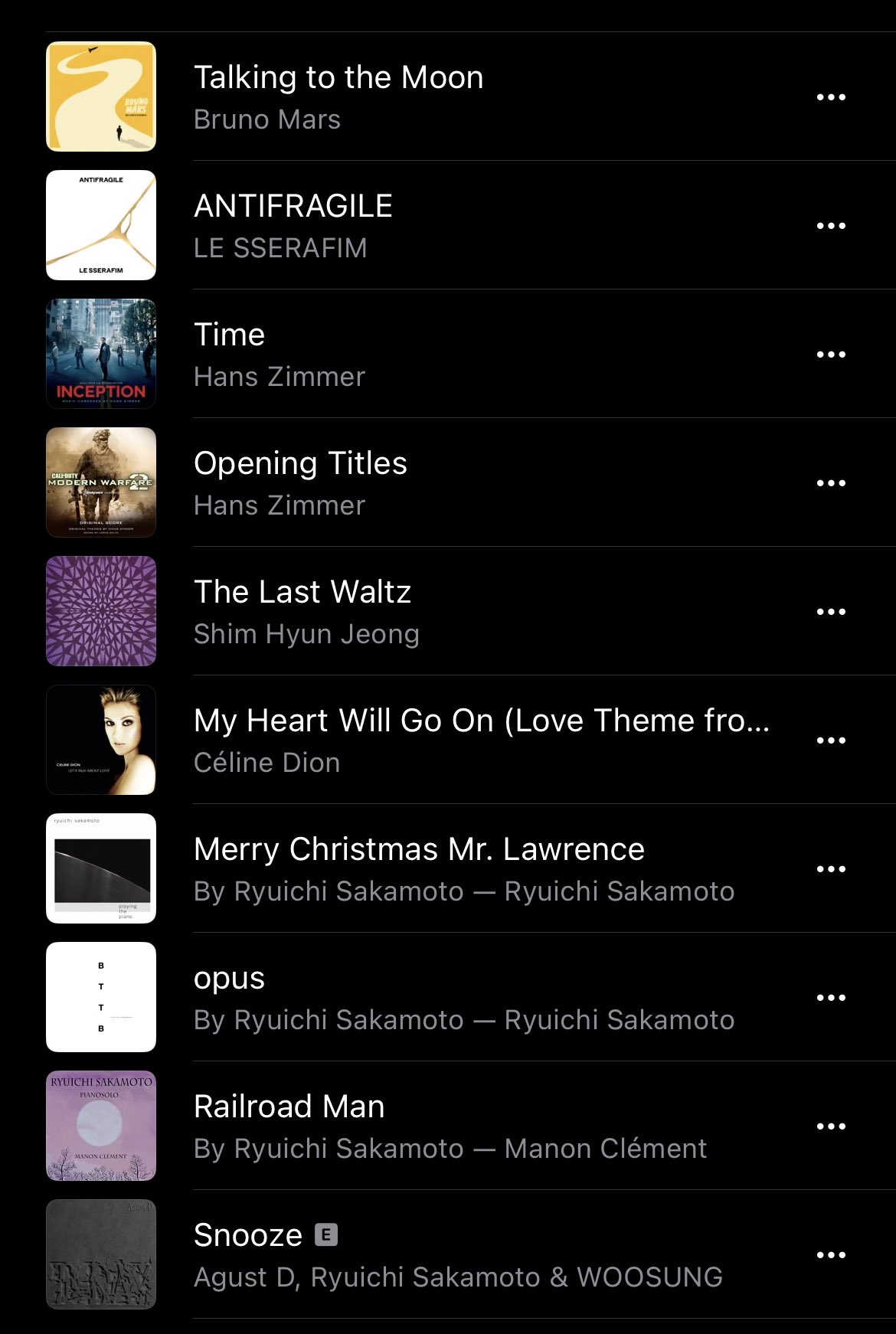The image captures a cell phone screen displaying the results of a music search on an aggregator site. The screen is predominantly black, creating a stark contrast with the content. On the left side, tiny square icons resembling album covers are aligned vertically. In the middle of the screen, song titles are displayed in bright white font, each followed by the artist's name in a slightly dimmer, off-white or gray font. For example, the first song listed is "Talking to the Moon" by Bruno Mars. On the extreme right, a column of three-dot icons is visible, indicating additional options or features accessible via drop-down menus. Ten different songs are featured on this page, though the specific search term is not evident from the display.